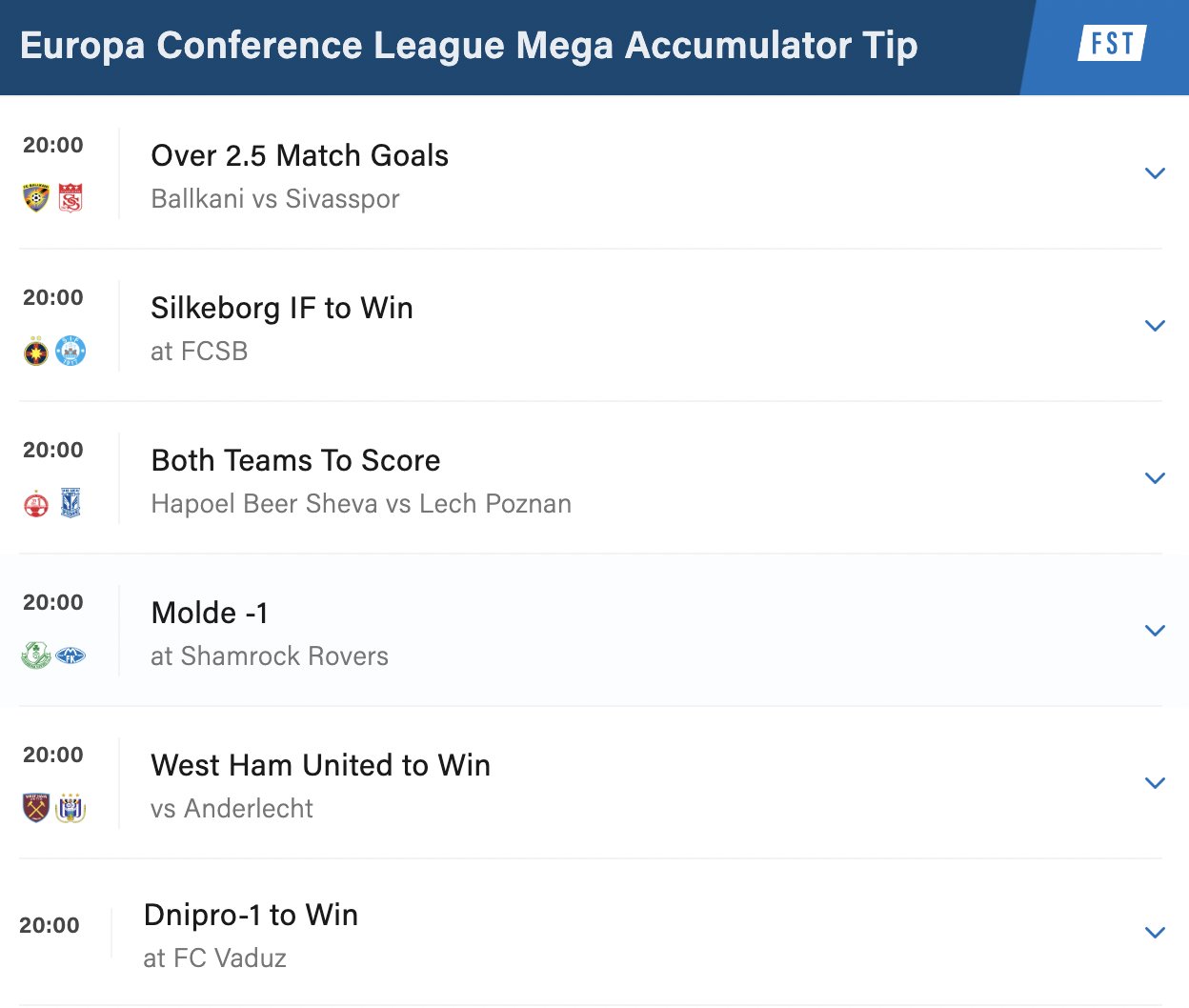This descriptive caption could be written as follows:

---

**Detailed Description of a Europe Conference League Mega Accumulator Tip Graphic:**

The graphic displays a Europe Conference League mega accumulator tip, set against a gradient background that fades from dark blue on the left to a lighter blue on the right. On the far right, there is a small rectangle featuring the letters "FST" prominently in blue.

At the top of the graphic, the title "Europa Conference" is written in a bold white font. Beneath this title, on a white background with black or gray text, the details of the accumulator are listed as follows:

1. **Balkani vs. Sivasspor**: Over 2.5 match goals scheduled at 20:00. 
2. **Silkeborg IF to Win at FCSB**: Match scheduled at 20:00.
3. **Hapoel Be’er Sheva vs. Lech Poznań**: Both teams to score.
4. **Molde to Win at Shamrock Rovers**.
5. **West Ham United to Win at Anderlecht**.
6. **West Ham United to Win at F.C. Vaduz**.

On the right side of each match entry, there are pull-down menu icons, suggesting that each selection can be expanded for further details.

---

This elaborative description should give a clear and detailed understanding of the graphic’s contents and layout.